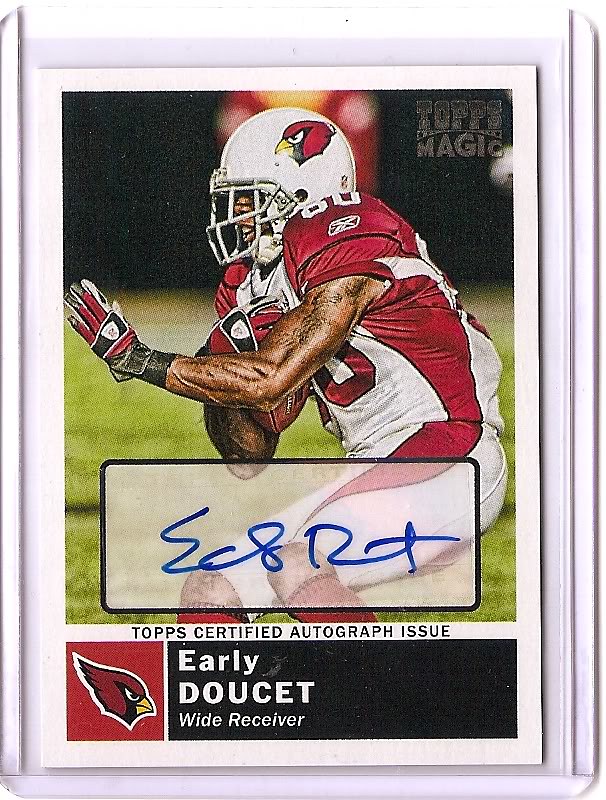This photograph showcases a Topps Magic football card of Early Doucet, a wide receiver for the Arizona Cardinals. The card is encased in a clear plastic protector and depicts Doucet in motion, clad in a red and white jersey numbered 80, with tattoos on his visible arm, and wearing a white helmet featuring an angry bird logo with a red head, black face, and yellow beak. Doucet is clutching a brown football against his chest with his gloved right hand, while extending his left arm forward. He sports a metal visor over his helmet and the Reebok symbol is visible on his red sleeve. The backdrop shows a green field. The card includes Doucet's blue ink signature within a black-outlined, semi-transparent white section. Below this section, on a white banner, it states "Topps Certified Autograph Issue" in black text. Adjacent to the banner is the Arizona Cardinals' red bird logo, and directly beneath that, in white letters on a black background, it reads "Early Doucet Wide Receiver." The card has a distinct aged look and is consistent with classic designs from Topps.